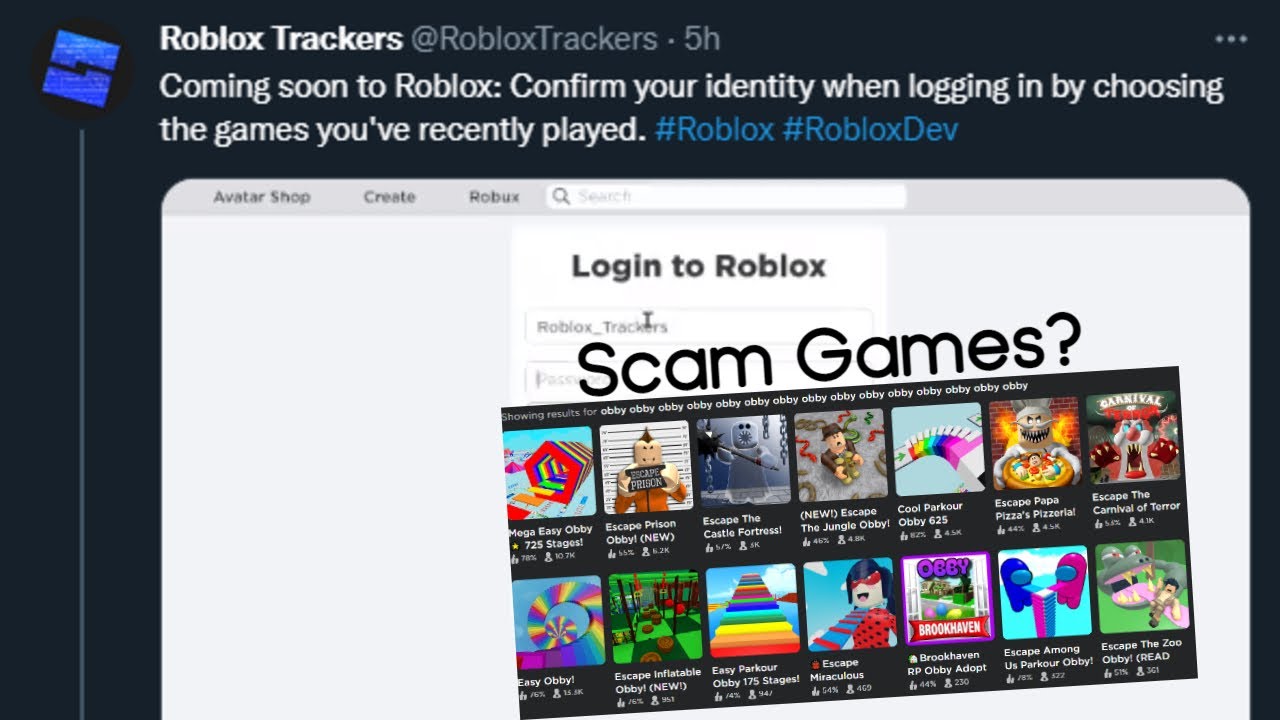This image displays a screenshot of a tweet from the Twitter account @RobloxTrackers, whose display name is also Roblox Trackers. The tweet was posted five hours prior to when the screenshot was captured. The tweet announces a new upcoming feature for Roblox, stating: "Coming soon to Roblox: Confirm your identity when logging in by choosing the games you've recently played. #Roblox #RobloxDev."

Attached to the tweet is an image illustrating the new feature. The image shows the Roblox sign-in screen with an additional layer displaying icons of various Roblox games. Some of the game titles listed include "Escape Papa Pizza's Pizzeria," "Escape the Carnival of Terror," "Escape Miraculous," "Easy Parkour Obby," "Easy Obby," "Mega Easy Obby," and "Escape Prison Obby." Each game is represented by its respective icon.

The profile picture of @RobloxTrackers is a blue Roblox logo.